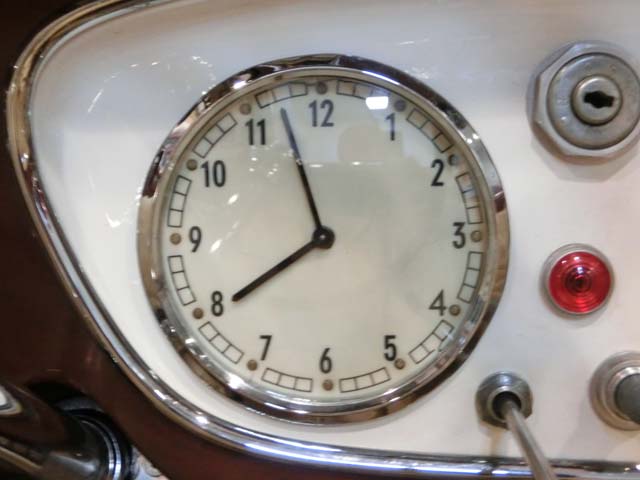A detailed and cleaned-up caption for the image could be:

"Photograph of a vintage car dashboard with an intriguing design. The dashboard features an ornate clock set to 7:55, showcased against a mother-of-pearl background and bordered by polished silver chrome. Below the clock, there is a toggle switch and two lights – one green and one red – providing functionality and a splash of color. The clock face potentially glows in the dark, adding an element of nocturnal elegance. An old-fashioned metal lock opening is positioned at the top, hinting at additional functionalities. The entire piece is oval-shaped, exuding an antique charm that harkens back to a bygone era of automotive design."